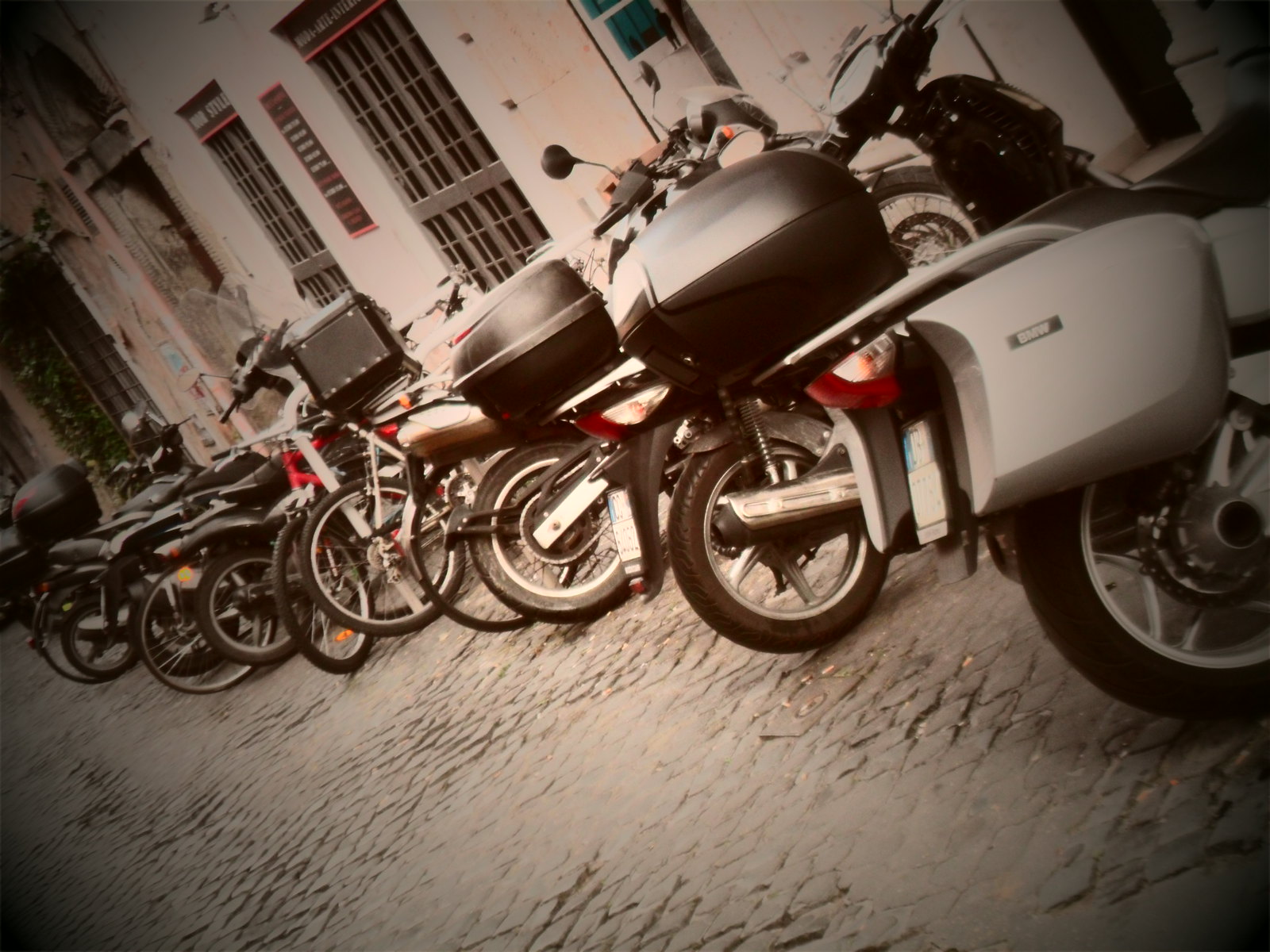This photograph, taken with a canted angle and a vintage sepia filter, vividly captures an outdoor scene full of character and a European ambiance. The foreground showcases a row of scooters, along with a few bicycles, all parked diagonally on an old, cobblestone street. The scooters, predominantly silver and black and equipped with carrying cases, are uniformly aligned from right to left, in front of a light-colored, smooth-walled building. The building appears to be a series of interconnected sections, possibly housing businesses or a restaurant, indicated by a barely legible sign that mentions "style." The architectural details include several doors, some with metal grates pulled down, suggesting they may be shops that are currently closed. The photo features a vignette effect that darkens the edges while keeping the center bright, emphasizing the charmingly weathered street and the stoic, neatly parked scooters.